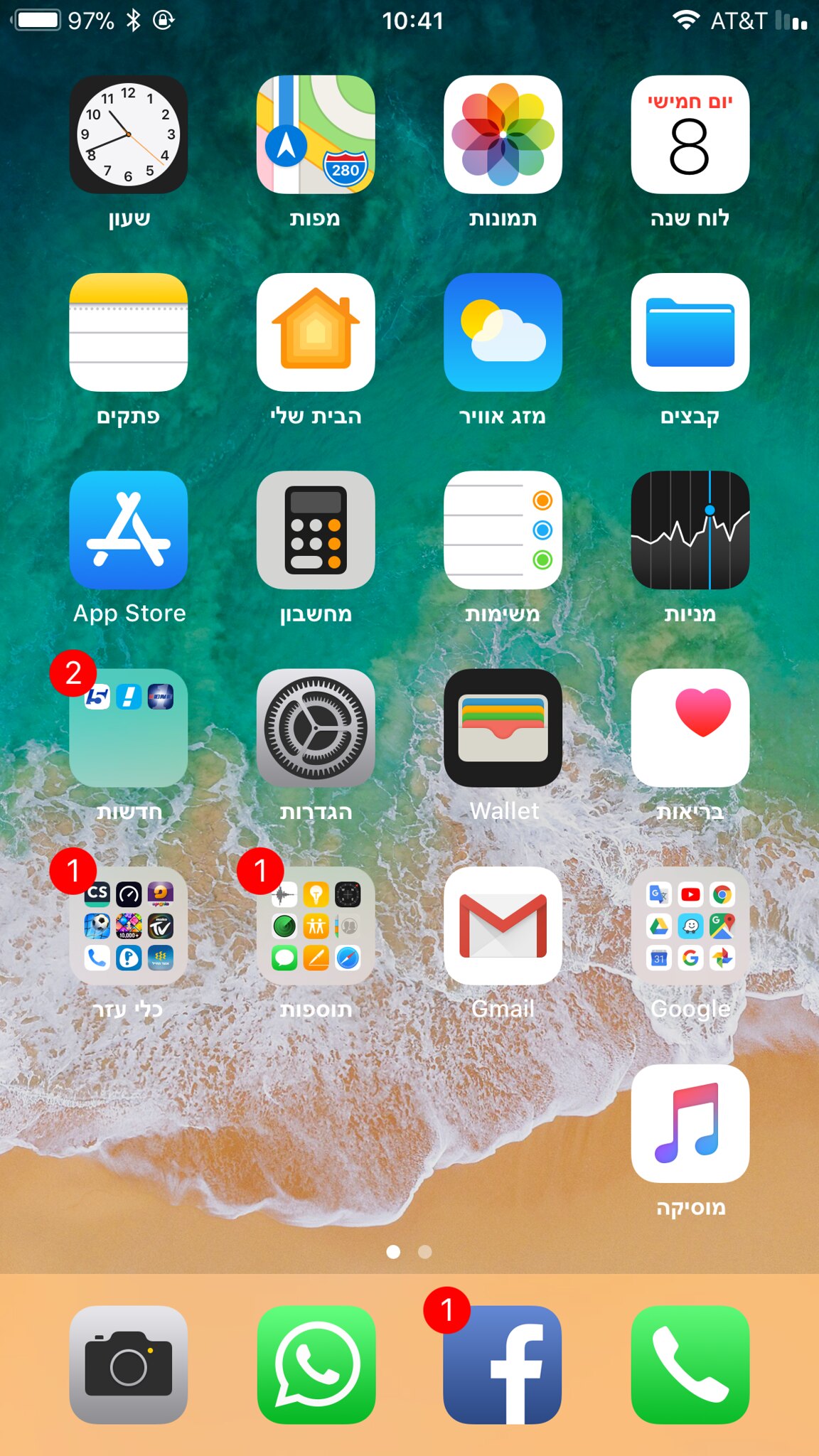This screenshot captures the home screen of an iPhone. The display shows the time at 10:41 AM, with the battery level at a healthy 97%. The phone is connected to the AT&T cellular network. 

Organized neatly in a grid, the screen features five rows of four app icons each, with a sixth row hosting the docked applications typically found at the bottom of an iPhone home screen. 

Starting at the top left, the following apps are arranged horizontally in the first row: Clock, Maps, Google Photos, and Calendar. The second row contains Notes, Weather, Files, and the App Store. The third row displays the Calculator, Reminders, Stocks, and an unidentified folder with three icons inside. Moving to the fourth row, you'll find Settings, Wallet, Health, and another folder with multiple icons. 

The fifth row consists of yet another folder with multiple icons, Gmail, another folder containing several icons, and the Google app. Beneath this, the pinned dock at the bottom of the screen includes Camera, WhatsApp, Facebook (showing one unread notification), and Phone.

Notably, some apps have names written in a different language, adding a touch of personalization and diversity to the user interface.